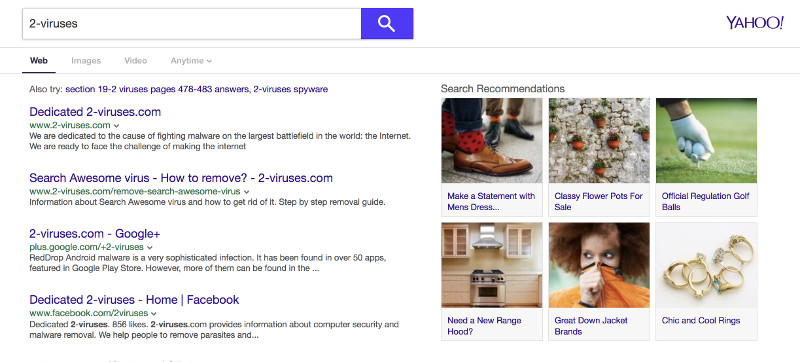A detailed caption for the image described:

The image displays a Yahoo search results webpage with a clean white background. Prominently, the word "Yahoo" is written in large blue letters at the top right corner of the page. On the left side of the page, there is a search box containing the text "two-virus." Adjacent to this box, on its right side, is a blue button featuring a magnifying glass icon.

Directly below the search box is a horizontal menu displaying several tabs: "Web," "Images," "Video," and "Anytime." Underneath this menu, within the "Web" tab, there is an "Also try" section suggesting the option "section 19.2 viruses page," highlighting various additional suggestions with numbers.

Further down, the main search results are listed vertically. The first result is titled "Dedicated to-two-virus.com." Following this, the second result reads "Awesome Virus Removal Guide," the third result links to "two-virus.com on Google Plus," and the fourth and final result is labeled "Dedicated to-two-viruses Home Page on Facebook."

Additionally, situated right below the top menu bar, there is a section labeled "Search Recommendations," featuring six small images. These images depict various items including men's shoes, flower pots, golf balls, rings, a jacket, and a range hood.